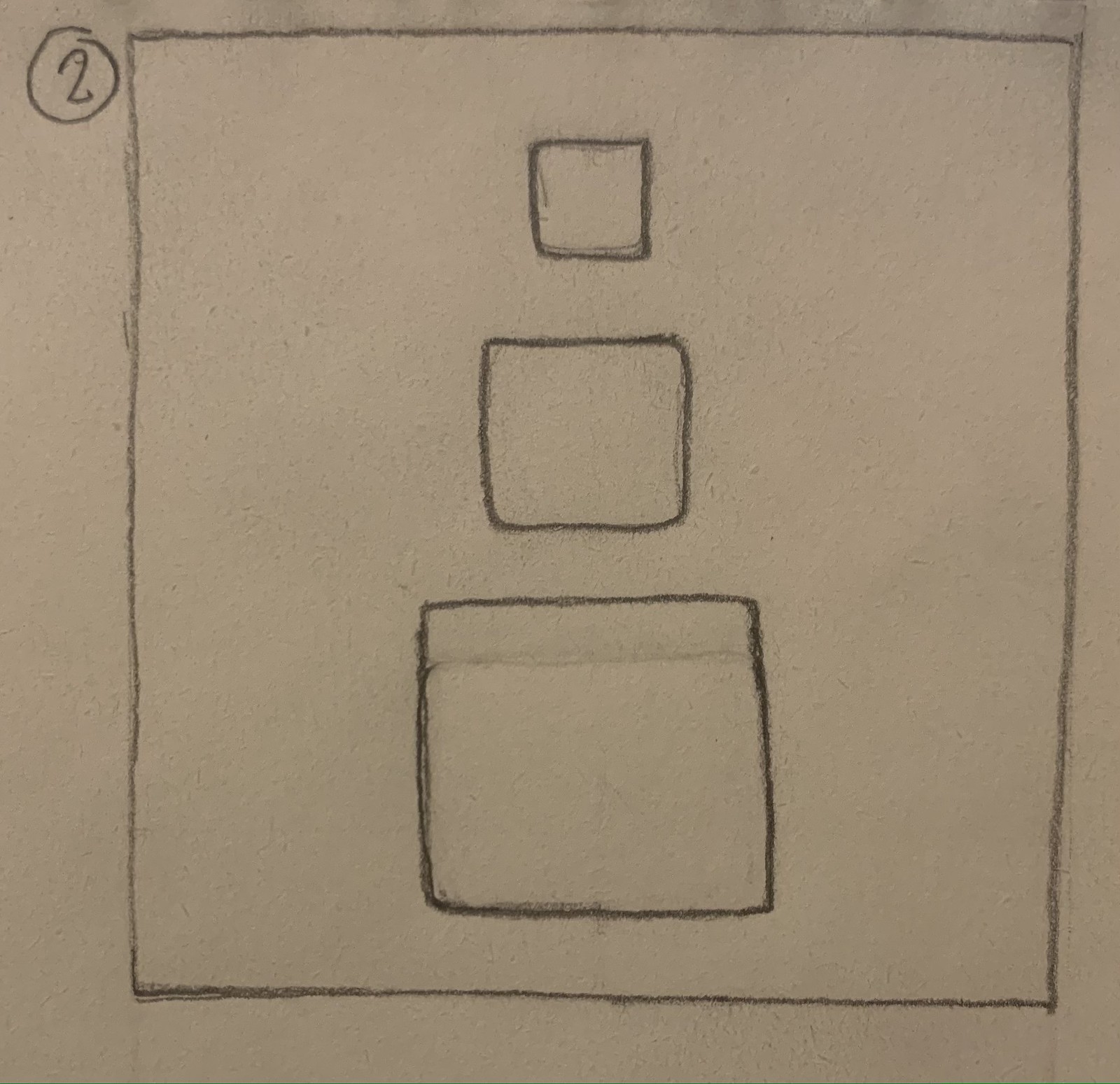On an off-white, slightly tan-colored sheet of paper, there is a meticulously hand-drawn diagram. In the upper left corner, a pencil-drawn circle almost completes its loop but falls slightly short, forming an incomplete circle. Inside this circle is the number "2." Adjacent to this is a square border, neatly encapsulating the main content of the drawing, suggesting this is "Box 2."

Inside the bordered area, there are three squares of varying sizes aligned vertically. The smallest square is at the top, followed by a modest gap of about an inch before the next, slightly larger square. Another inch of space separates this from the third and largest square at the bottom. Notably, about an inch down from the top of the largest square, there is a faint, partially erased line, hinting at prior adjustments to the drawing.